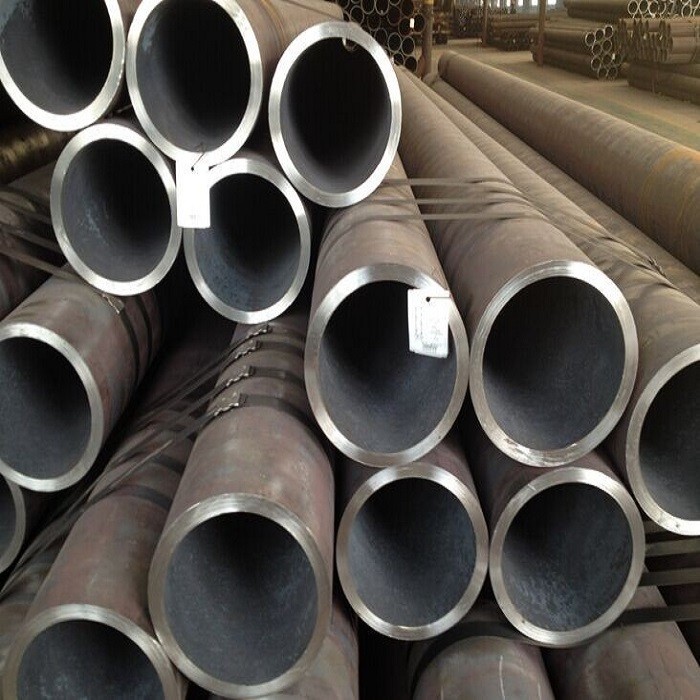The image depicts the interior of a warehouse dedicated to storing and possibly manufacturing tubing or large metal poles. In the foreground, there's a pile of approximately 10 to 15 dark gray to dark silver steel pipes, each roughly 10 to 15 feet in length and about 5 to 12 inches in diameter. These pipes are organized in groups and bound together with metal straps at the front and rear, resembling a log pile. Tags are attached to some but are not legible. The warehouse interior features a hard floor and extends quite a distance back into the frame, where additional stacks of similar pipes are visible. The entire scene is dominated by these metallic tubes, suggesting a storage or staging area for future projects. The overall color palette includes shades of gray, silver, black, and hints of white and green, indicating an industrial setting with adequate daytime lighting.